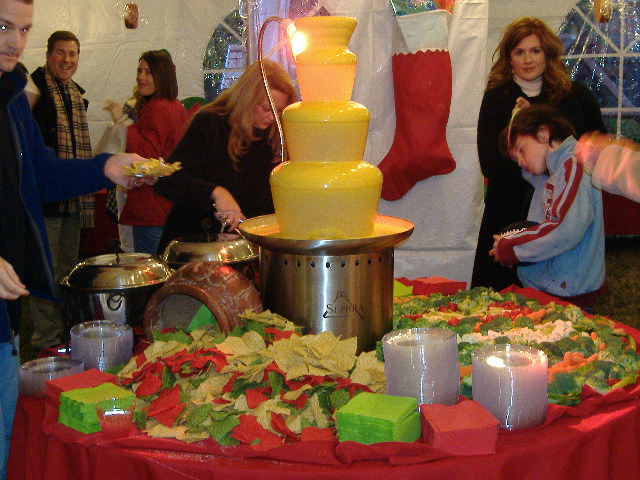This vibrant and festive image captures a bustling Christmas celebration, centered around a striking four-tiered cheese fountain. Positioned on a table adorned with a red tablecloth, the fountain flows into a gleaming stainless-steel pot. The table is lavishly decorated with red, yellow, and green tissue paper, which enhances the holiday atmosphere, along with an assortment of multicolored tortilla chips, green and red napkins, paper plates, and crudités featuring broccoli, carrots, cauliflower, and cherry tomatoes. 

On the right-hand side, a woman in a black jacket, holding her son dressed in a blue jacket, gazes directly at the camera. Between them and the group on the left, a red Christmas stocking hangs on the wall behind the table. The left side shows a man in a blue jacket holding a plate of nachos already dressed with cheese, while a woman behind him, also in a black jacket, uses her right hand to scoop food onto her plate. Behind them, a laughing couple poses for the camera. A disembodied arm extends into the frame from the left, hinting at more activity out of sight. The scene is set against a backdrop of a white wall, rounding out this lively moment at what appears to be an outdoor event hosted inside a large tent.